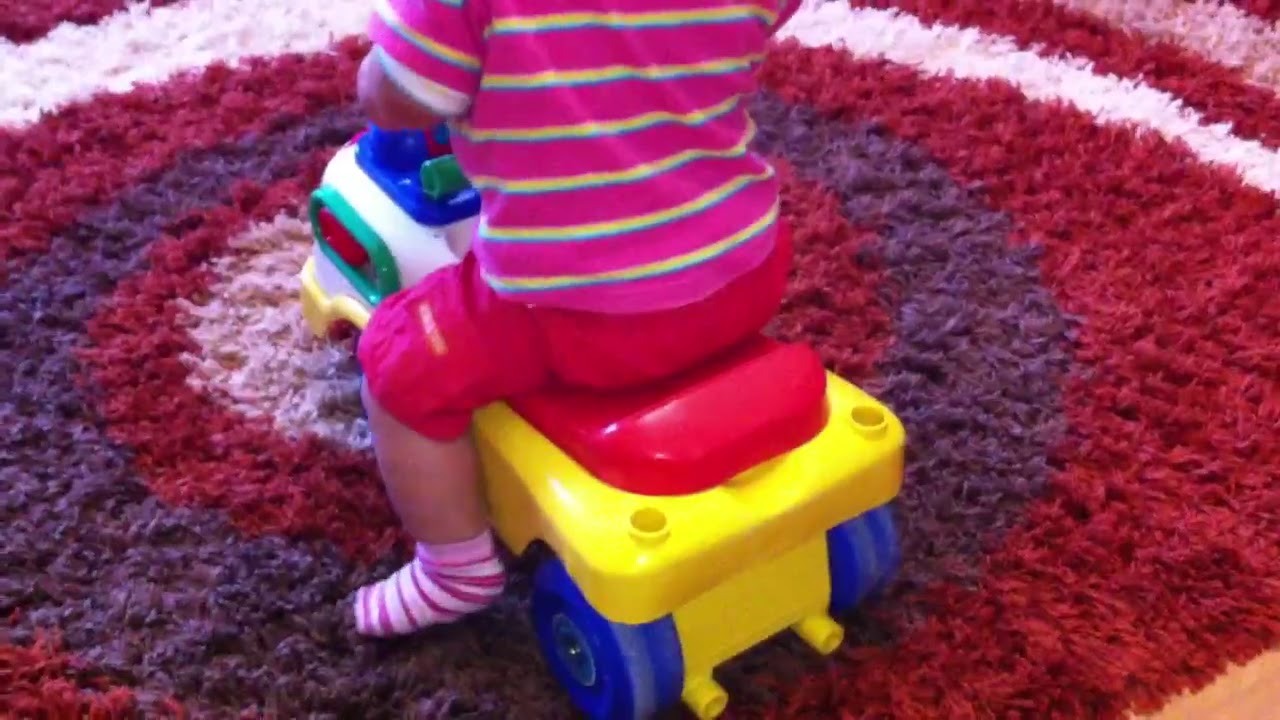This vibrant indoor photograph captures a playful moment of a child enjoying a colorful toy vehicle. Captured from the shoulders down and facing away from the camera, the child wears a bright pink shirt with yellow and blue stripes, dark pink pants, and pink and white socks. The ride-on toy features a yellow body, a red seat, blue wheels, and green accents, adding to the cheerful scene. The child is seated on a carpet with striking circular concentric patterns in white, red, and dark blue, enhancing the lively atmosphere of the setting.